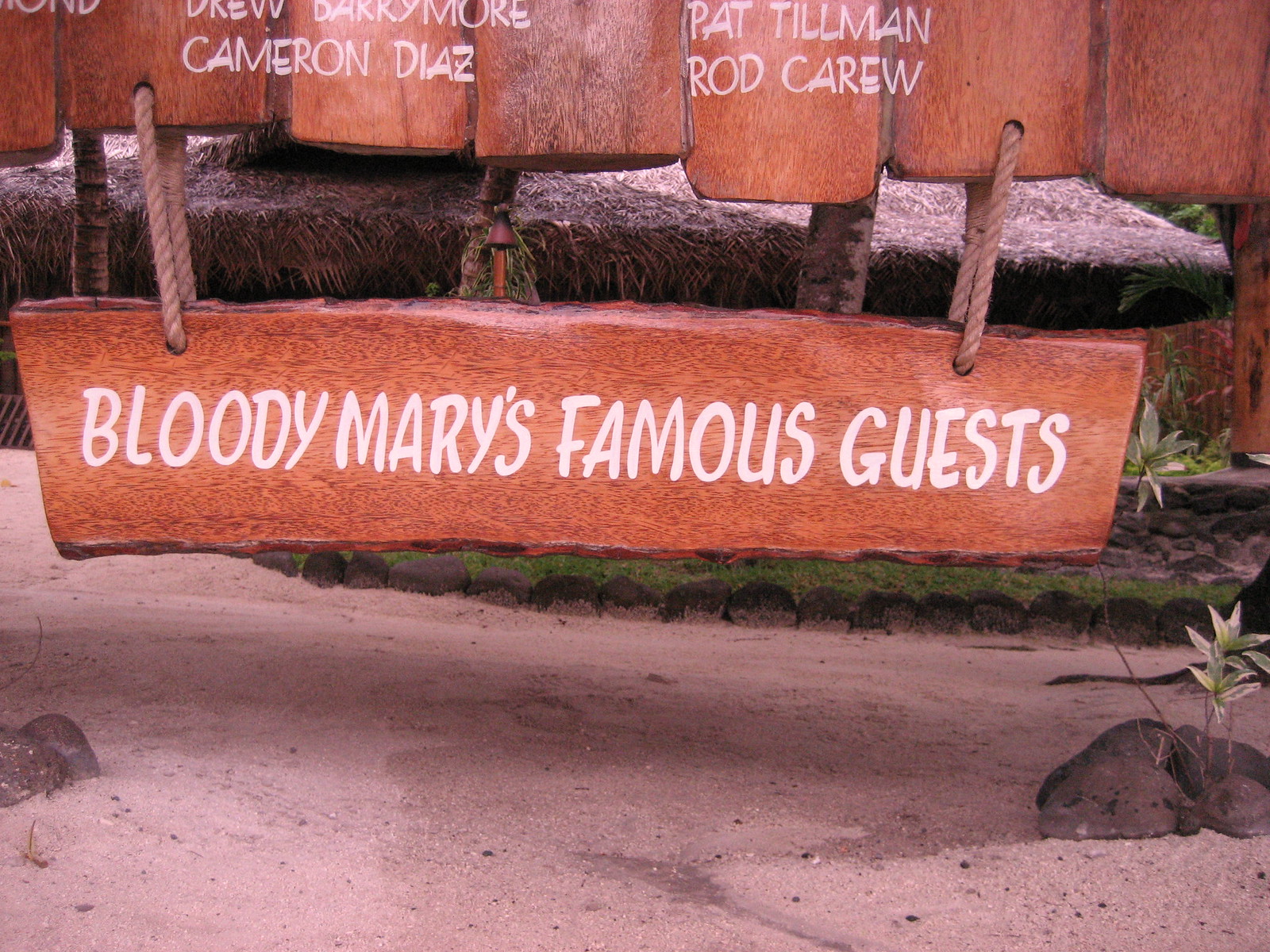The image depicts a public display featuring a long, glossy, brown wooden sign hanging from a beige rope. The sign, which has a smooth and shiny finish, is suspended from vertical wooden planks that appear to form the lower edge of a fence. The prominent white text on the sign reads “Bloody Mary's Famous Guests,” with the names Drew Barrymore, Cameron Diaz, Pat Tillman, and Rod Carew listed above it. Additional names are partially visible but cut off at the edge of the image. Beneath the sign lies a mixture of sand, gravel, rocks, and small plants, including a notable cluster of leaves emerging from the rocks in the lower right corner. The overall scene is devoid of people and is set against a backdrop of rocky terrain with sparse grass.